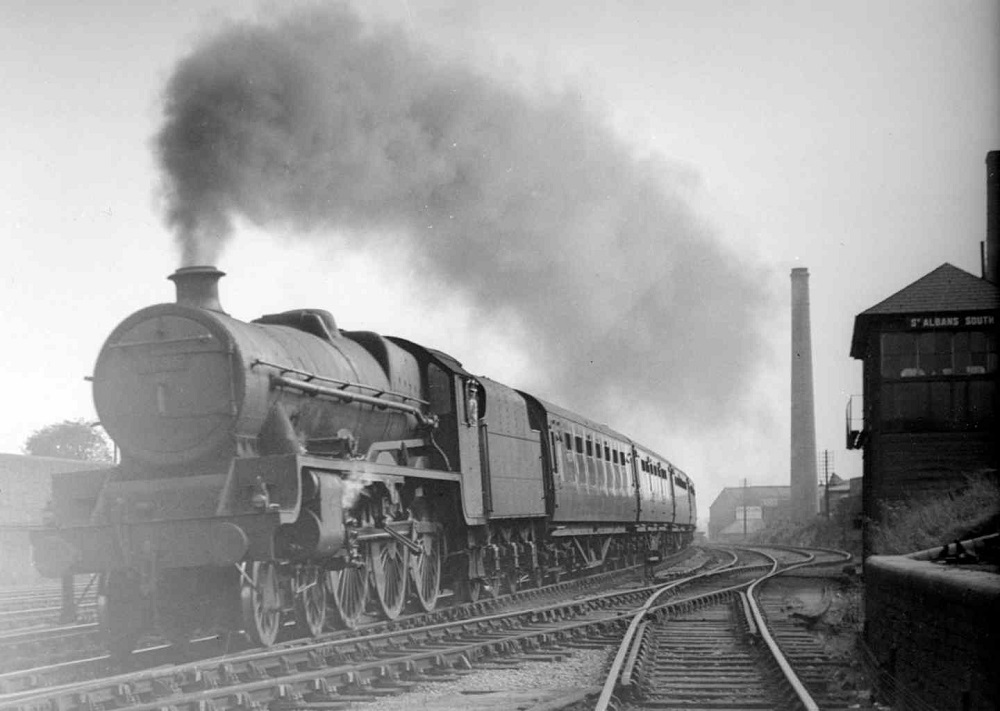This black-and-white photograph captures a vintage scene from what appears to be the early 20th century or even earlier. The perspective places the viewer directly on the train tracks, facing an oncoming, antiquated train characterized by its mechanical design and lack of modern amenities like extensive windows. The locomotive at the forefront is billowing thick smoke from its smokestack, which is indicative of its age and steam-powered nature. The train stretches back along the horizon, disappearing into the distance, with several passenger cars trailing behind it. This scene unfolds in what seems to be an old train yard, featuring multiple sets of tracks that diverge and intersect. Surrounding the train yard are a mix of tall and squat buildings, some of which appear to be constructed from brick or wood. One of these structures bears the name "Albans" along with other indiscernible text. The photograph, steeped in historical ambiance, encapsulates the industrial essence of a bygone era.